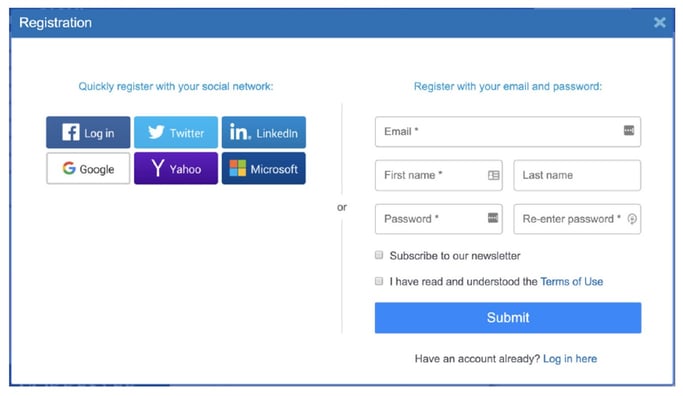**Detailed Caption:**

The image features a pop-up registration menu on a website bordered in blue. At the very top, there is a blue bar with white text. The bar is labeled "Registration" on the left, and on the right, it includes a clickable "X" button to close the pop-up.

Below this blue bar, the pop-up contains a white rectangular section divided into two halves. The left side starts with blue text that reads, "Quickly register with your social network:". Underneath, there are two rows of social media icons for quick registration: the top row includes icons for Facebook, Twitter, and LinkedIn from left to right. The bottom row features icons for Google, Yahoo, and Microsoft.

The right side of the pop-up comprises a classic email registration form. It has fields to input your email, first and last name, password, and a re-enter password for confirmation. There are also checkboxes to opt into subscribing to the newsletter and agreeing to the terms of use. Finally, at the bottom of the form, there is a "Submit" button to complete the registration process.